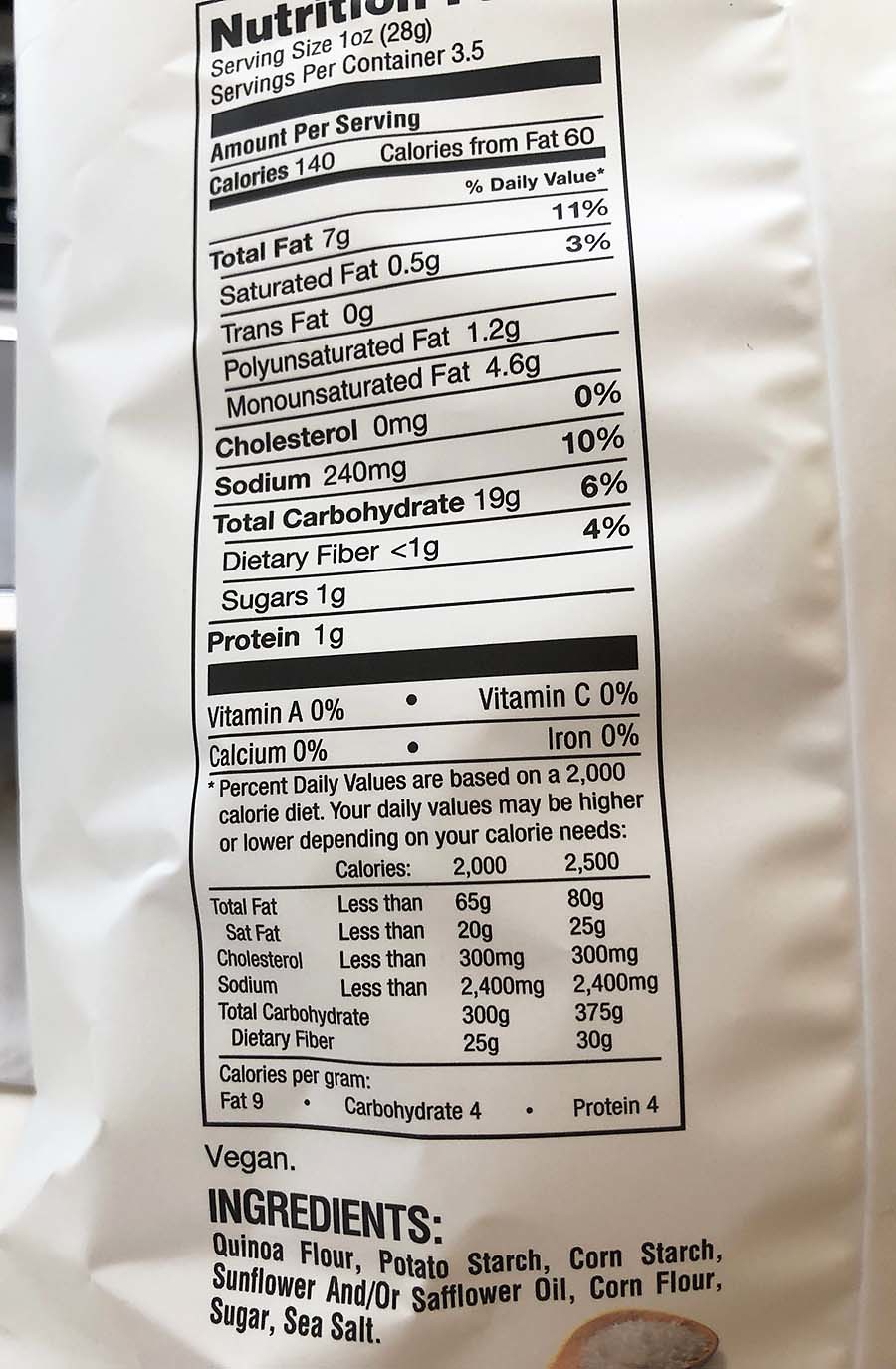This image displays the nutritional information and ingredients list of a food product, likely a type of quinoa-based chip, although the exact item is unclear. The primary ingredient is quinoa flour, followed by potato starch, cornstarch, sunflower and/or safflower oil, corn flour, sugar, and sea salt. According to the nutritional facts, each serving size is 1 ounce, and the package contains approximately 3.5 servings. Per serving, the product contains 140 calories, 7 grams of fat, 0 milligrams of cholesterol, 240 milligrams of sodium, 19 grams of carbohydrates, and 1 gram of protein. The image does not provide enough visual context to definitively identify the product, but the ingredients and nutritional content suggest it is a quinoa chip or a similar snack.